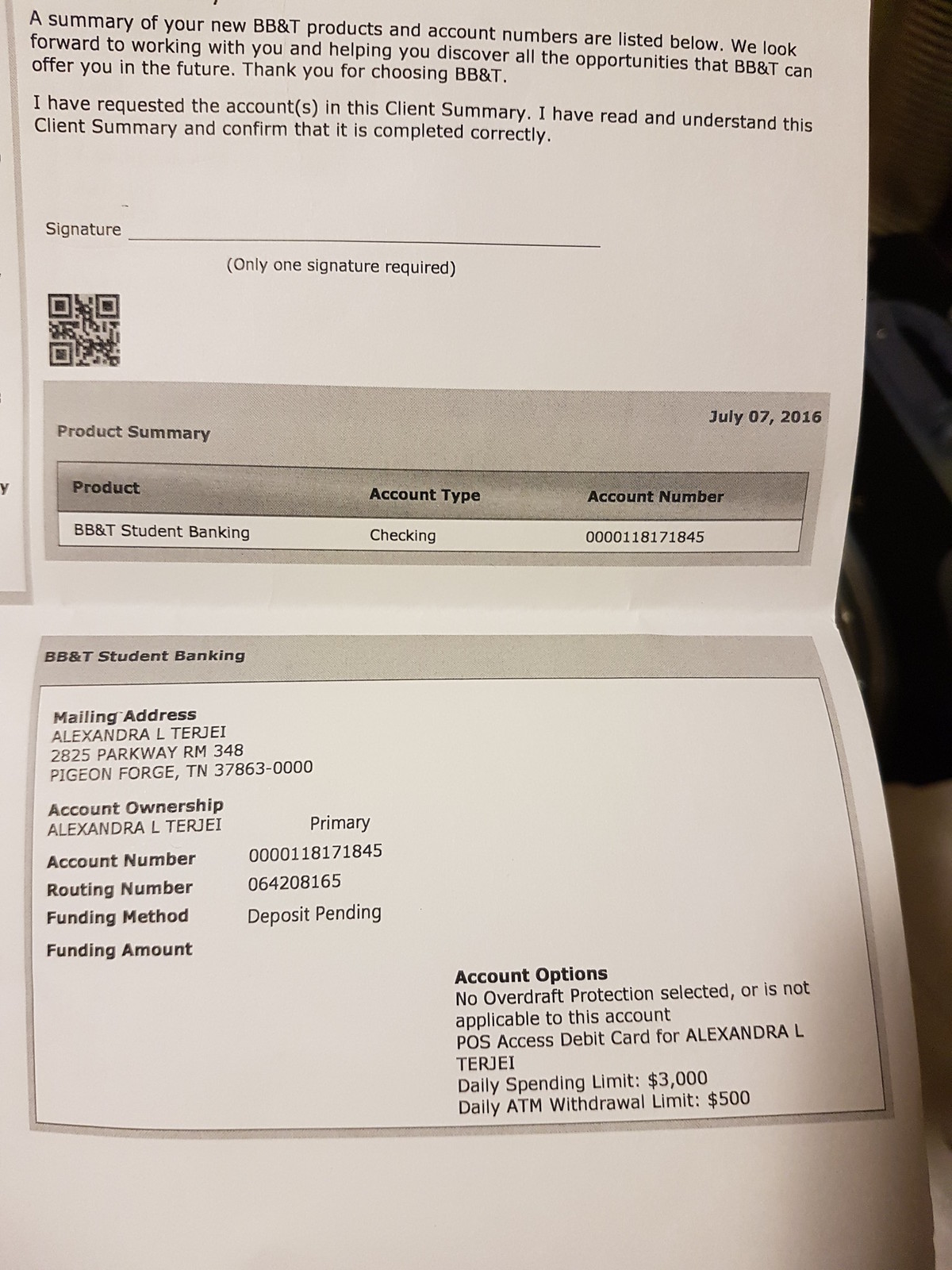The image is a close-up color photograph of an official document resembling a bank statement or invoice from BB&T, prominently featuring a white piece of paper with a noticeable crease down the middle. The header of the document reads "A summary of your new BB&T products and account numbers are listed below. We look forward to working with you and helping you discover all the opportunities that BB&T can offer you in the future. Thank you for choosing BB&T." Below this affirmation, the document has a space for a client confirmation with text stating, "I have requested the account in this client summary. I have read and understood this client summary and confirmed that it is completed correctly," followed by a blank signature line that specifies "only one signature required." Beneath the signature line, there's a QR code, followed by a gray text box that dates the document to July 7, 2018. The detailed section underneath includes a brief product summary mentioning "BB&T Student Banking," the account type as checking, and partial mailing address information of an individual named Alexandra, residing in Pigeon Forge, Tennessee. Additionally, there are small, barely readable lines that include personal data such as account and routing numbers. The photograph also captures elements of its surrounding environment; along the right side, there are other objects and items visible on what appears to be a desktop or table surface with hints of blue in the background.